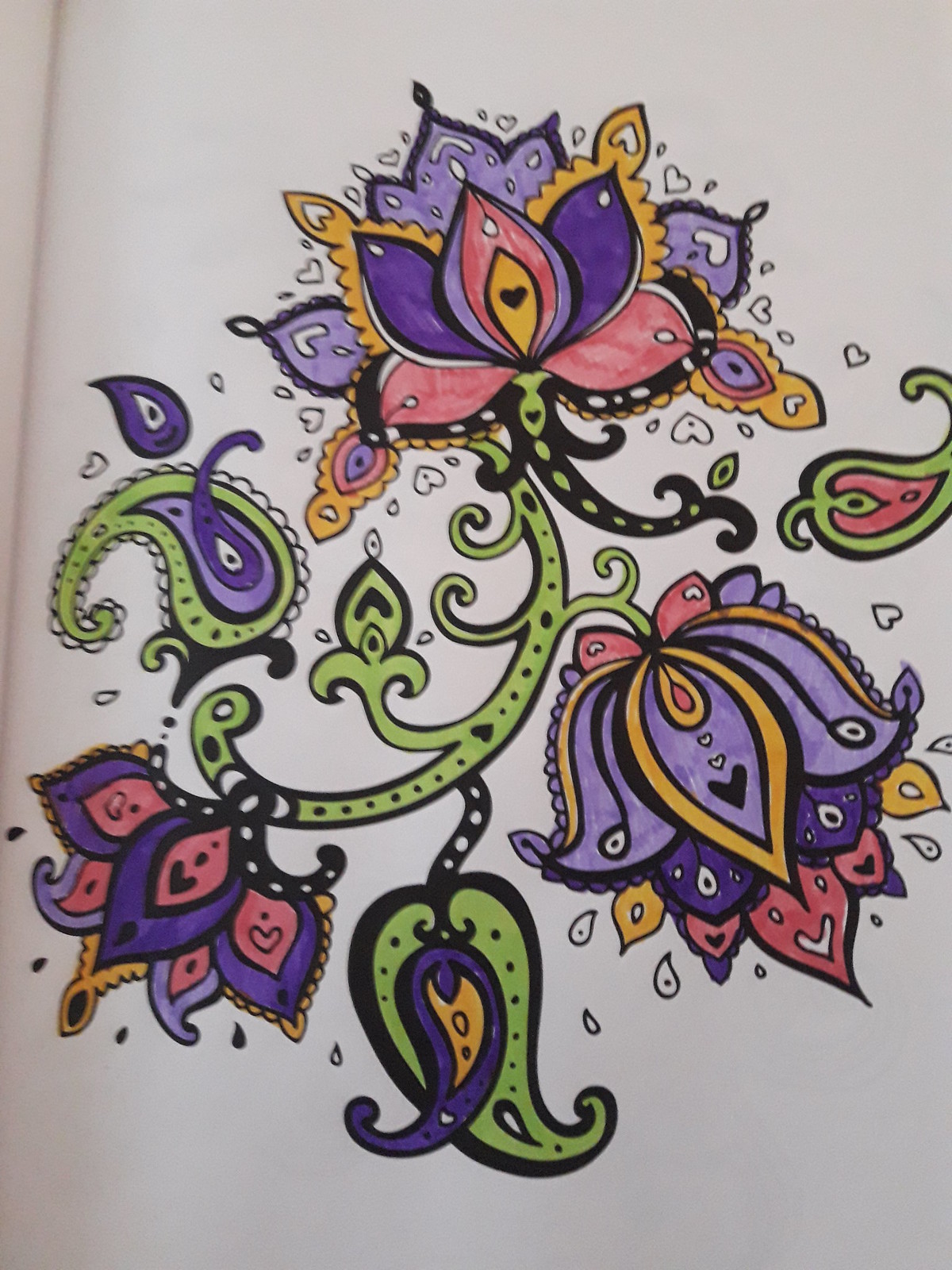This photograph captures a vibrant piece of artwork sketched on a crisp white page of a sketchbook. The drawing, rendered in thick black lines with black pen, features a lotus flower in a tattoo-inspired abstract style. The stems and leaves are shaded in green felt-tip pen, while the petals burst with hues of purple, pink, and yellow. Adding an element of whimsy, small heart shapes encircle the flower, and one of the petals is uniquely adorned with a smiley face that incorporates a heart motif. The detailed line work and dynamic colors make this artwork particularly striking and imaginative.